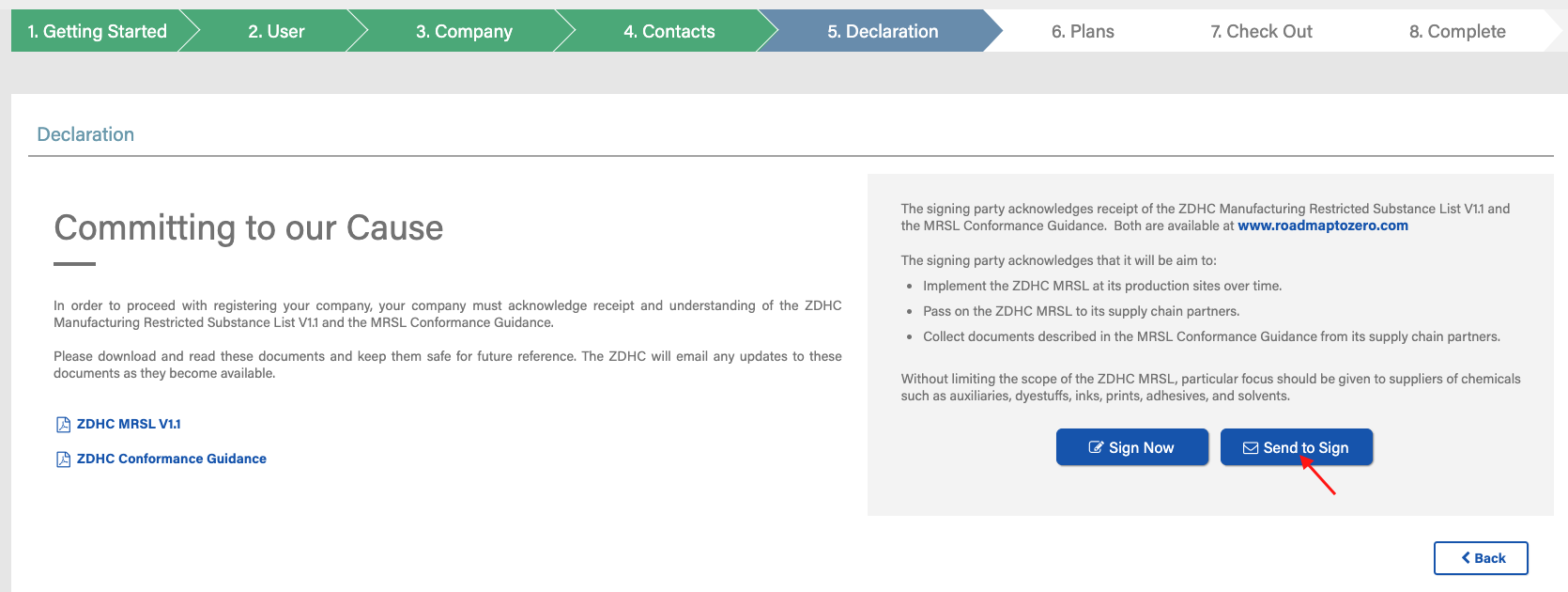The image showcases a "Declaration" page from a registration process. At the top of the page, a thin rectangular navigation bar features eight tabs, each separated by a white arrow-shaped divider. The first four tabs have a green background with white text: "1. Getting Started," "2. User," "3. Company," and "4. Contacts." The fifth tab, highlighted in blue with white text, reads "5. Declaration." The remaining three tabs are labeled "6. Plans," "7. Checkout," and "8. Complete," all in white text against a neutral background.

Directly beneath this navigation bar lies a gray horizontal band that reads "Declaration," serving as a visual separator from the rest of the content below. The content area is split into two sections: a white left side and a gray right side. On the left, the text "Committing to Our Cause" appears, with an underline emphasizing the "C" and "O." Below this title, a statement outlines that to proceed with the company registration, the company must acknowledge receipt and understanding of the ZDHC Manufacturing Restricted Substance List.